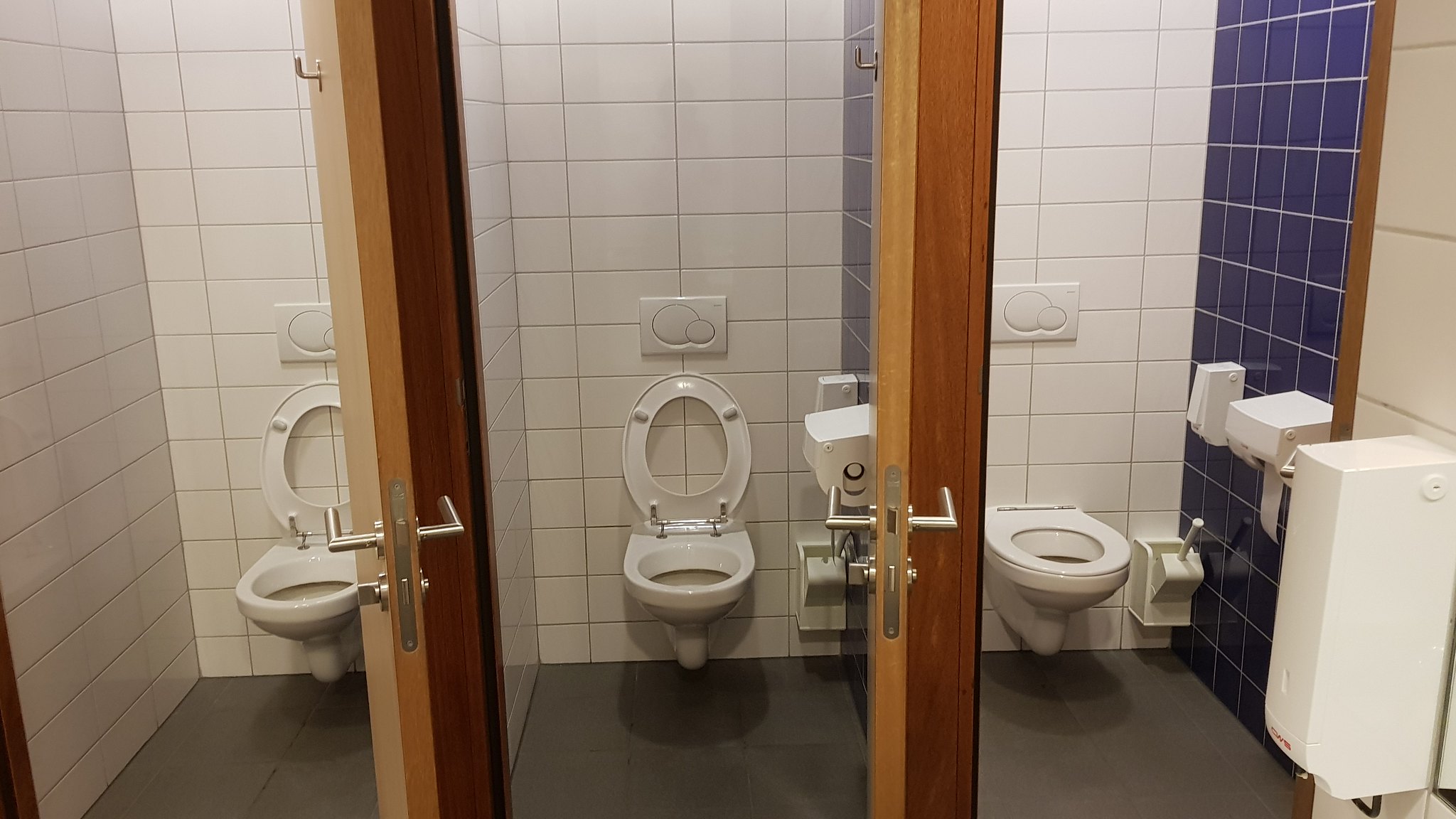This photograph captures the interior of a bathroom with three separate stalls arranged horizontally. Each stall is equipped with a white toilet, and the doors to all stalls are open, revealing their contents. The doors appear to be light wooden with silver handles. The left and middle stalls have their toilet seats raised, while the rightmost stall has a toilet without a seat. Mounted above the toilets are dual flush buttons, featuring a large circle for a full flush and a smaller circle for a half flush.

The stalls are divided by tiled walls; the left and middle stalls have white rectangular tiles on the back and left walls, while the right-hand stall features the same white tiles on the back wall and dark blue tiles on the right wall grouted with white. Each stall contains a toilet paper dispenser: the left and middle stalls on the right wall near the toilet, and the right stall has its on the left wall. Both the middle and right stalls also have a toilet brush with a white handle positioned in a holder on the lower right side. 

The flooring of the bathroom is covered in gray laminate. On the wall to the right of the stalls, there is a long rectangular dispenser, likely for paper towels or soap, mounted on white tiles. The overall design suggests a practical, clean, and functional space.